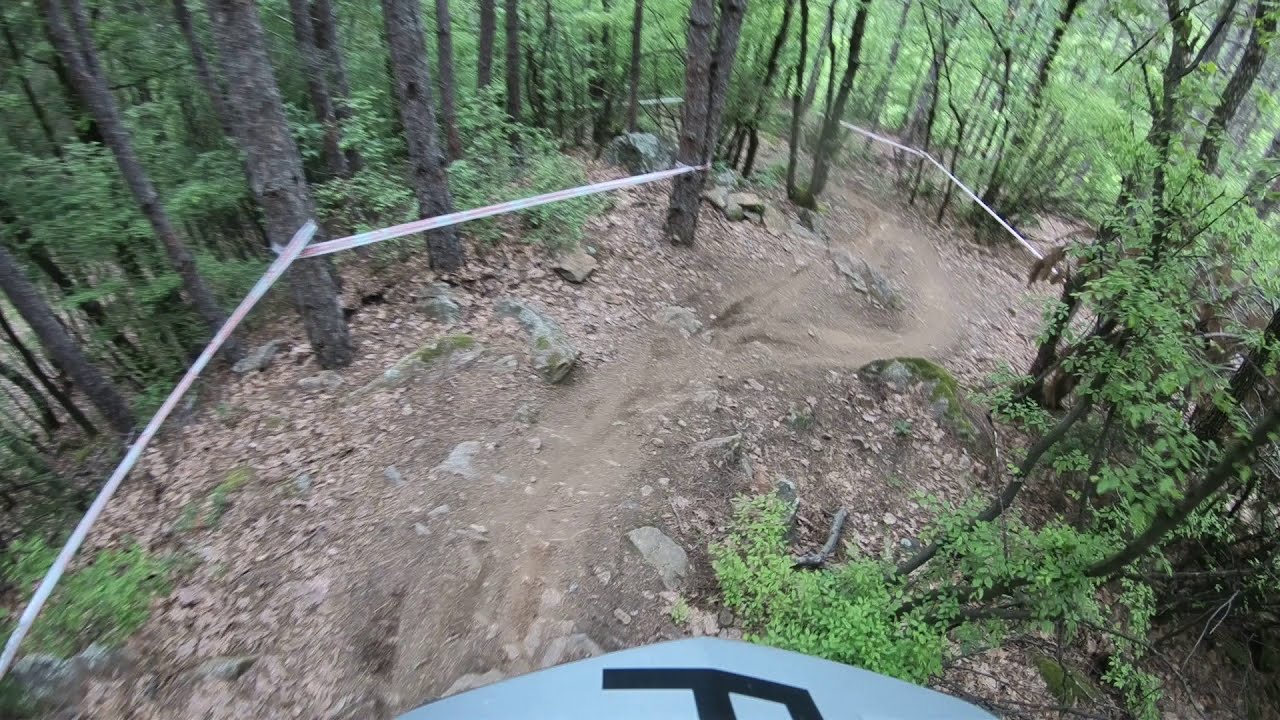The image depicts a steep, winding trail in a dense forest, predominantly featuring green deciduous trees with some pines. The forest floor is a mix of brown dirt, dead leaves, and a few bushes. The trail, likely designed for mountain biking or possibly dirt biking, is marked by white nylon tape wrapped around thin tree trunks on either side, indicating the path's direction. At the bottom center of the image, partially cut off, there is a gray, triangular object with a black marking, likely the top of a helmet or a part of a bike, suggesting the involvement of some type of off-road vehicle. The scene captures a rugged, downhill course through the natural, verdant surroundings.